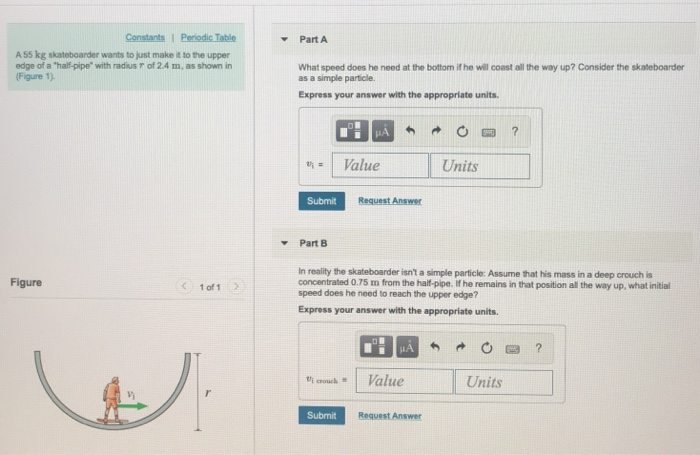The image is a blurred, light gray computer screenshot featuring a diagram and written instructions likely related to a physics problem. Dominating the left side is a blue rectangular section labeled "Constants and Periodic Table." Below it, text describes: "a 55 kg skateboarder wants to just make it to the upper edge of a half pipe with a radius of 2.4 meters as shown in figure 1." The diagram shows the skateboarder at the bottom of the half pipe. Towards the bottom on the left, it says "Figure 1 of 1."

On the right side, the image contains more instructions, divided into two sections. At the top right, labeled "Part A," it asks, "What speed does he need at the bottom if he will coast all the way up? Consider the skateboarder as a simple particle." Below this text, there is a blank rectangular field where an answer can be input, followed by a "Submit" button and a "Request Answer" option. Similarly, at the bottom right, another set of instructions is labeled "Part B," indicating an additional question or extension to the problem described in Part A.